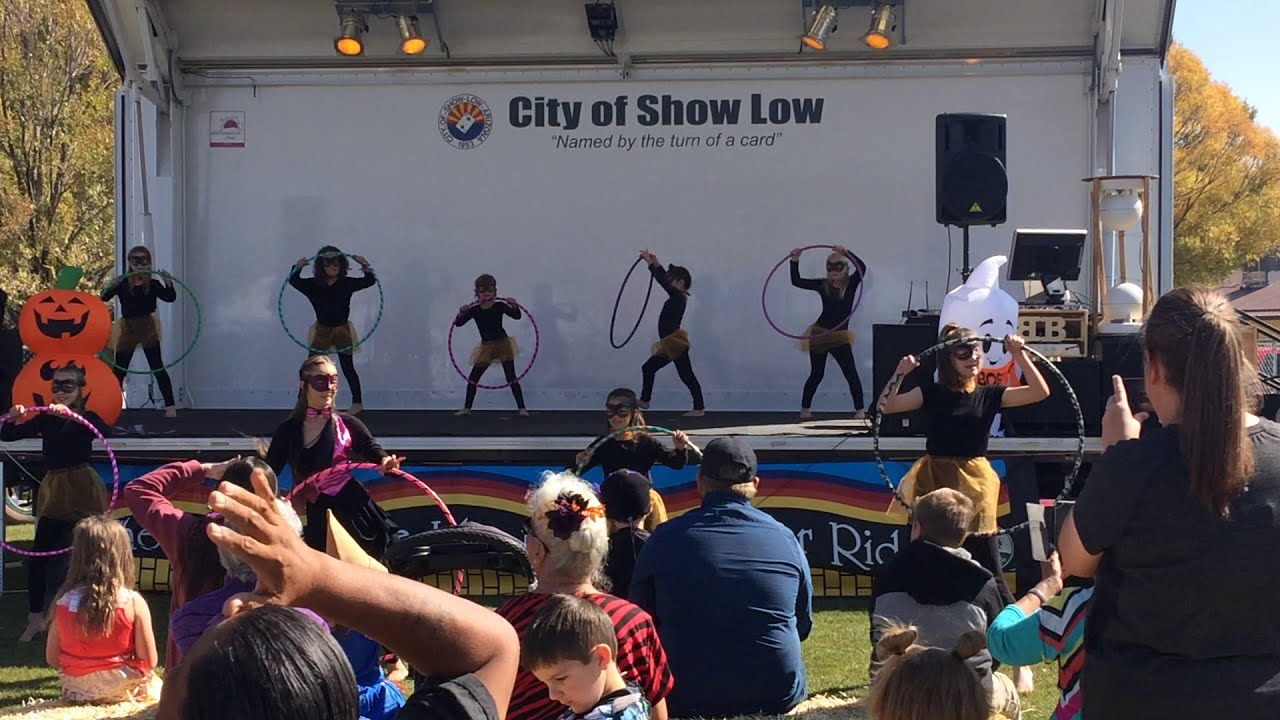The image captures an outdoor city event in Show Low, highlighted by a banner that reads "City of Show Low, Named by the Turn of a Card." The focal point is a group of young performers, likely dressed for a Halloween-themed performance. They wear black tops and tights with orange skirts, complemented by black eye masks, engaging in a hula hoop routine. The stage, embellished with a colorful, rainbow-like banner, features double-decker pumpkin decorations on the left and what appears to be a Casper-the-ghost decoration on the right. The event is well-lit with four strobe lights illuminating the performers. Below and in front of the stage, some dancers continue their hula hoop routines on the grass, amidst a diverse audience seated on the ground. This audience comprises individuals of various ages and races, some intriguingly holding their hands on their heads as they watch the performance.